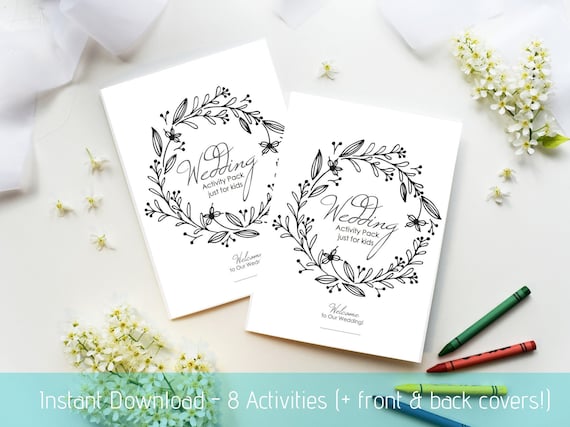This promotional photograph, taken from a top-down perspective on a white fabric background, features two wedding activity packs designed for children. Each pack is styled as a white card adorned with a black-and-white wreath of leaves and flowers on the cover. 'Wedding' is prominently displayed in elegant cursive in the center of each card, with 'Activity Pack Just For Kids' written underneath in a non-cursive font. Further down in cursive, 'Welcome' is scripted, followed by 'To Our Wedding' again in non-cursive. At the bottom of the cards, a digitally added light blue overlay bar reads 'Instant Download - 8 Activities (Plus Front & Back Covers)!' in white font. Complementing the cards, four crayons in green, red, yellow, and blue are arranged on the bottom right, and delicate sprigs of white flowers with yellow centers appear in the top left and bottom left corners of the photo.